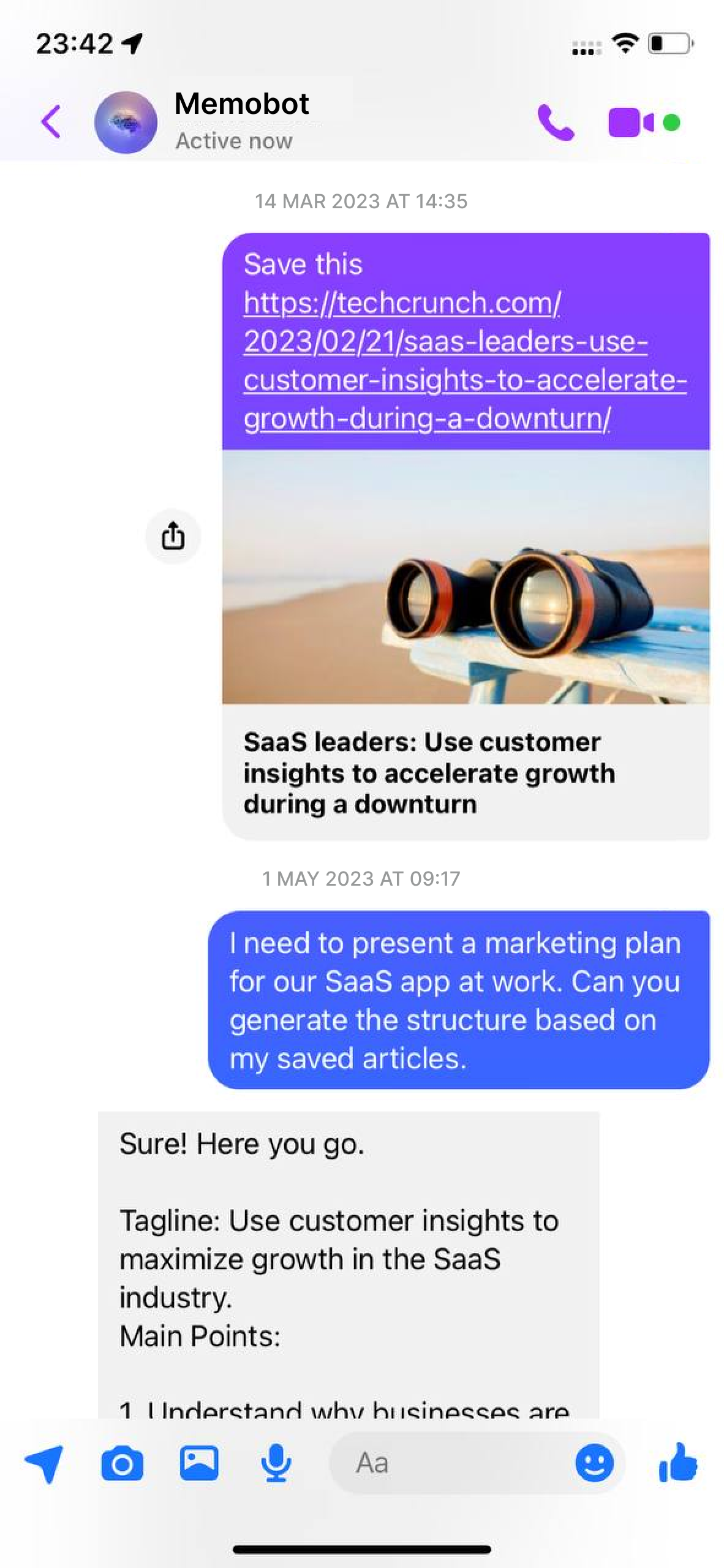A detailed screenshot of a chat interface from a phone:

At the very top of the screenshot, there is a light gray banner showing the device's status bar. On the left side, the time is displayed as "23:42." Next to the time, a location icon is present, followed by the signal service indicator showing three out of four bars. Further to the right, the Wi-Fi signal icon is visible, and the battery icon, partially filled with black, indicating its current charge level, sits at the far right end.

Below the status bar, a purple left-pointing arrow is seen, which is used to go back. Adjacent to it is a circular purple avatar representing 'MemoBot,' with the name "MemoBot" written in black and capitalized as "MemoBot." The status "active now" is indicated in gray text next to the name. To the right of "MemoBot," there is a purple phone icon and a purple camera icon (for video chat) with a green circle in front of the camera icon.

The chat background is white, with messages primarily displayed within this area. A timestamp in gray reads "14 of March, 2023 at 14:35." Below it, a message starts with a purple link preview. The top half of the preview is purple, with white text saying "save this," followed by a URL link to TechCrunch. The preview shows part of an article with the headline, "SaaS leaders use customer insights to accelerate growth during a downturn," visible in gray text beneath the URL.

An image within the message preview shows a picturesque beach scene: a blue, cloudy sky and brown sand. A white table is also seen, with a pair of black binoculars resting on it. The binoculars feature an orange ring around the lens, which reflects the sunny sky.

A subsequent message is timestamped "1st of May, 2023 at 09:17," displayed in a blue speech bubble with white text: "I need to present a marketing plan for our SaaS app at work. Can you generate the structure based on my saved articles?" 

Following this, there’s a gray box containing a reply from 'MemoBot' in black text, beginning with "Sure, here you go," followed by: "Tagline: Use customer insights to maximize growth in the SaaS industry. Main points: 1. Understand why businesses are..." The rest of the message is cut off, indicating that more content follows in the chat.

At the bottom of the screenshot, several icons appear: a blue arrow, a blue camera, a blue picture icon, a blue microphone, and a gray formatting bar showing "A" and "a" in gray letters. Additionally, a blue smiley face and thumbs-up icon are present, with a black half-arrow also visible halfway up the screen.